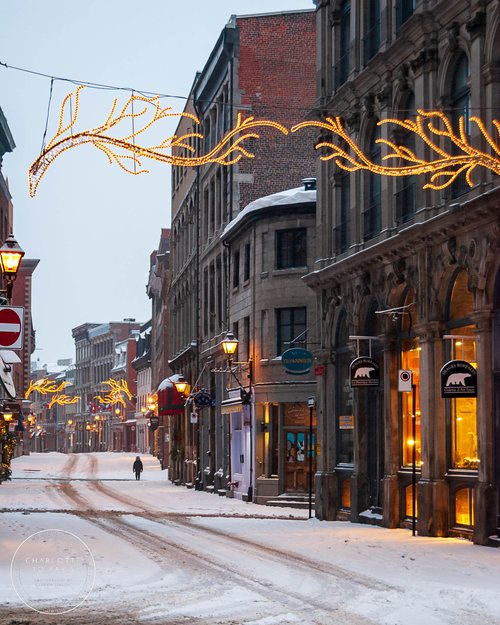This photograph captures a serene winter scene on a wide, snow-covered street in what appears to be an older, possibly foreign town or a mid-20th century setting. The street, seemingly empty save for a lone pedestrian, features tire tracks running down its center amidst light snow cover. Both sides of the street are lined with approximately four-story tall buildings, among them a notable department store on the left with illuminated windows and a sign featuring a polar bear. Across the street, other brick buildings stand adorned with small Christmas lights, adding to the festive atmosphere. Strings of golden, lit-up Christmas decorations resembling tree branches and antlers stretch across the street from the electric lines above, illuminating the scene right down to the distant street lights. The sidewalk appears well-trodden, and the overall setup evokes a nostalgic, small-town American northeastern vibe, possibly with a population around 100,000.